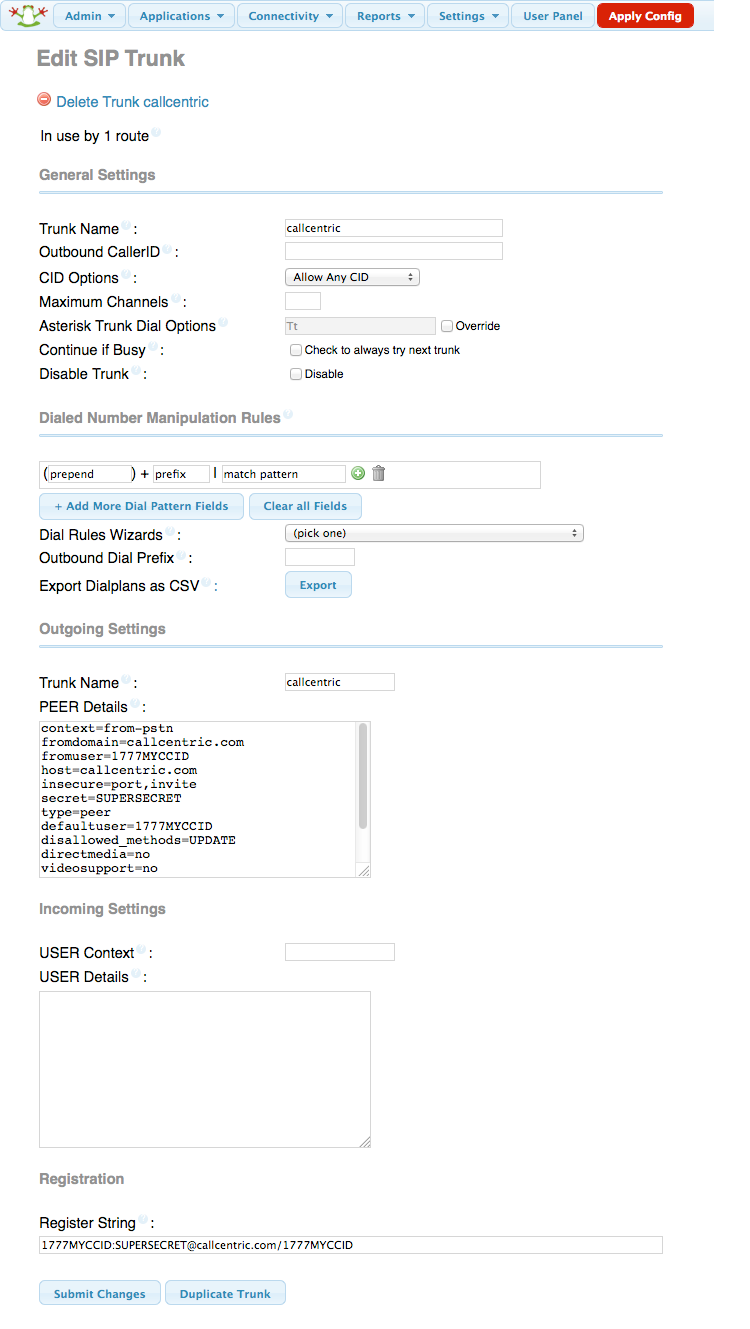**Descriptive Caption:**

The image depicts a user interface of an administrative settings page for managing SIP trunks in a telecommunications application. The page features a white background with text in black, red, and blue colors. Various elements include:

- Text descriptions and labels.
- Several drop-down menus for options and configurations.
- Categories listed on a sidebar to the left: Admin, Applications, Connectivity, Reports, Settings, User Panel.
- Main operational buttons for "Apply Configuration", "Edit SIP Trunk", and "Delete Trunk Call Centric".
- A detailed section for general settings, including fields for "Trunk Name" (set to "call centric") and "Outbound Caller ID". 
- Configuration options such as "CID Options" (set to "Allow Any CID"), "Maximum Channels" (currently not filled), and "Asterisk Trunk Dial Options" with an option "CT" (Continue if Busy) which includes a check box to "Always Try Next Trunk" and an option to "Disable" it.
- Additional sections include "User Contexts", "User Details" (both containing empty fields), and "Registration" with a specific "Registration String".
- At the bottom of the page, there are two input fields and buttons labeled "Submit Changes" and "Duplicate Trunk".

The interface design combines functionality with a straightforward layout to enable effective telecommunication management.